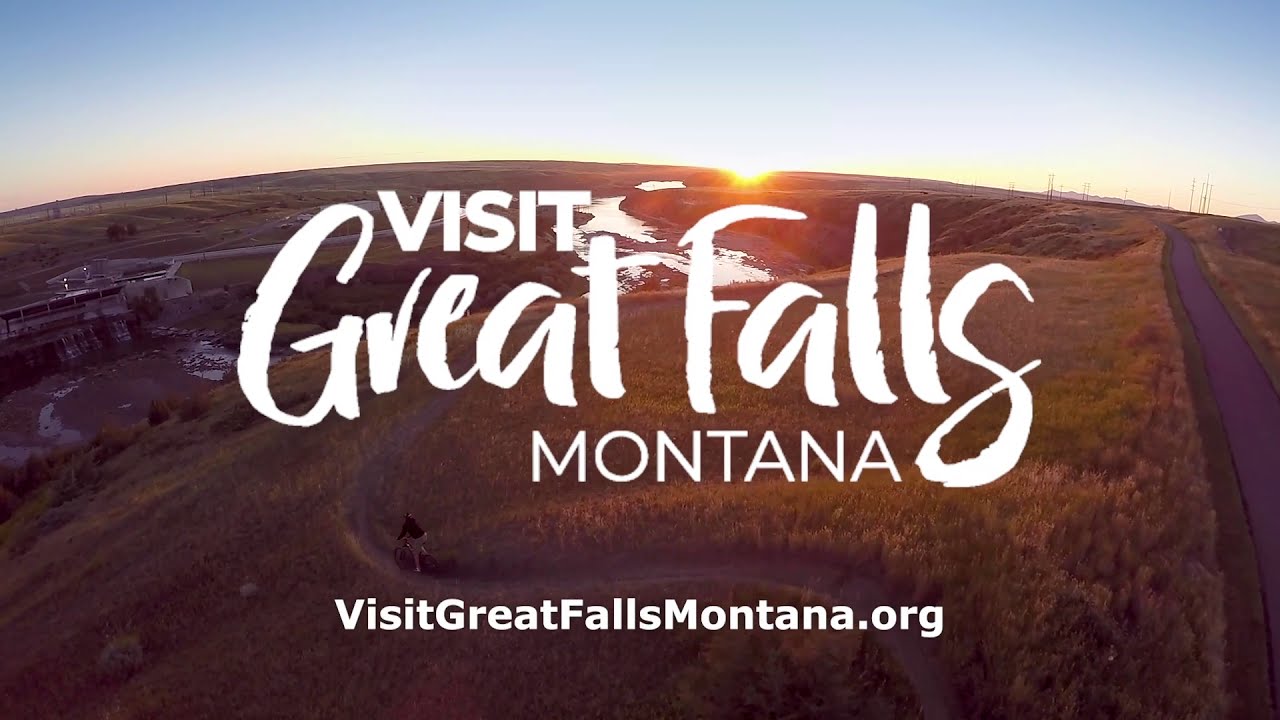The advertisement features a stunning aerial view of Great Falls, Montana. The landscape comprises expansive, flat grassy fields, with a partially visible dirt path meandering through the center. A lone cyclist, dressed in black and beige, navigates the winding trail. To the right, a country road stretches off into the distance. The sun is tenderly setting, casting an orange and blue hue across the sky and highlighting the serene water body and the fenced areas within the scene. On the far left, a solitary building punctuates the vast openness of the horizon. Superimposed text in the center of the image reads, "Visit Great Falls, Montana," with a URL at the bottom, visitgreatfallsmontana.org, inviting viewers to explore the natural beauty and tranquility of Montana.